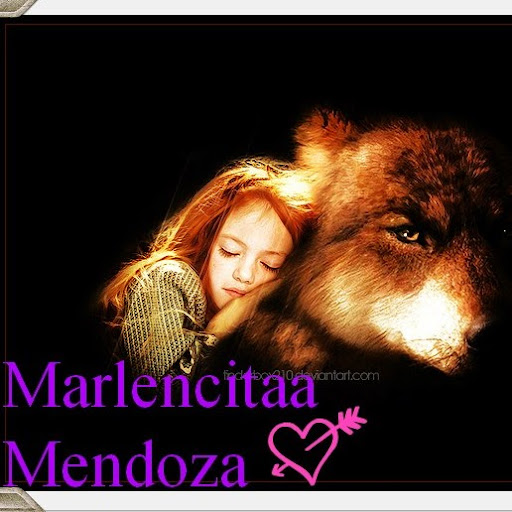The image features a serene young girl with long ginger hair and a pale complexion, clad in a gray top. She is depicted with her eyes closed, leaning gently against the neck of a brown bear adorned with brown eyes, adding a sense of peacefulness to the scene. Set against a flawlessly crisp black background, the image carries a sense of intimacy and tranquility. In the bottom left corner, the name "Marlencita Mendoza" is inscribed in purple text alongside a small pink heart with an arrow piercing through it, resembling a logo. There's also a mention of a divine art website, suggesting that this unique and potentially digitally altered artwork could serve as a movie poster or promotional material.